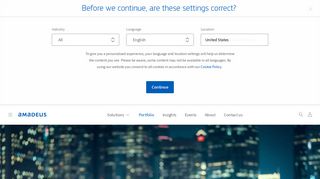This image appears to be a small and somewhat blurry screenshot taken from a computer screen. The image lacks a defined border and features a dialog box at the top with blue text reading, "Before we continue, are these settings correct?" Below this question are three input fields: the first labeled "All," the second presumably showing "English," and the third indicating "United States." Beneath these fields, there is an area of tiny, unreadable black text. In the center of the image, there is a blue rectangular button labeled "Continue." 

On the left side, the text "Amadeus" is displayed in blue, and it seems that the user has clicked on a word that looks like "Portfolio," also colored in blue. Underneath this, a wide rectangular image spans the width of the screen, depicting a nighttime cityscape with numerous buildings illuminated by lights. The scene is dark and somewhat blurry, conveying a bustling urban environment.